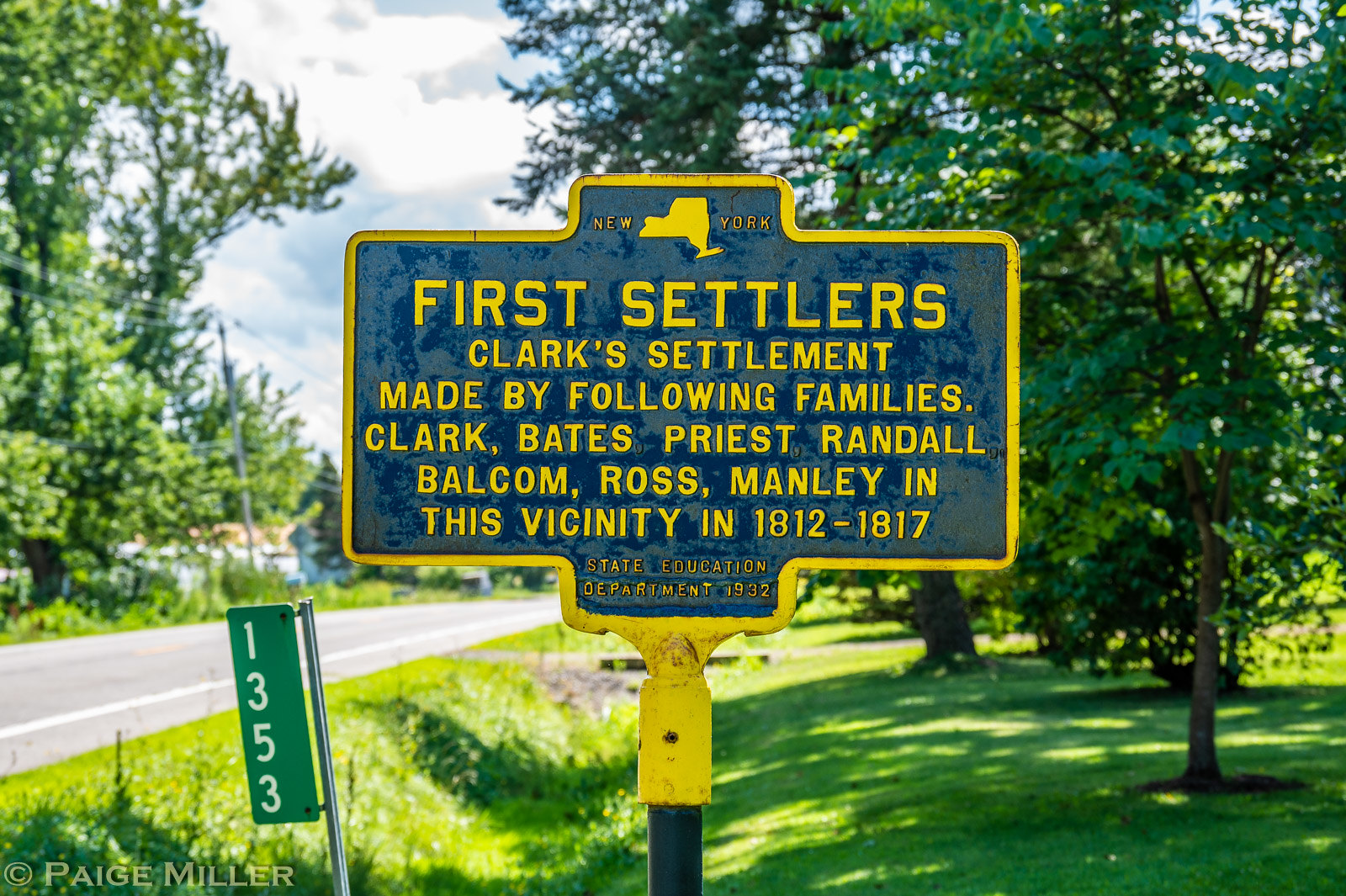The photograph captures a historical marker set into a black metal pole, situated outdoors beside a road. The metal plaque has a yellow painted border and a blue background, featuring yellow raised lettering. The top center of the sign has the word "New York" along with an outline of the state. The main text reads: "First Settlers Clark Settlement made by the following families: Clark, Bates, Priest, Randall, Balcom, Ross, Manley in this vicinity in 1812-1817. State Education Department 1932." The plaque exhibits visible signs of aging, with rust particularly prominent around the edges, where it connects to the pole. Behind the sign, a grassy lawn with multiple large trees adorned with green leaves stretches out, while a mile marker with the numbers "1-3-5-3" on a green background stands to the left. The scene also includes power lines, additional trees, and a cloudy sky, highlighting the historical marker's picturesque yet weathered setting.